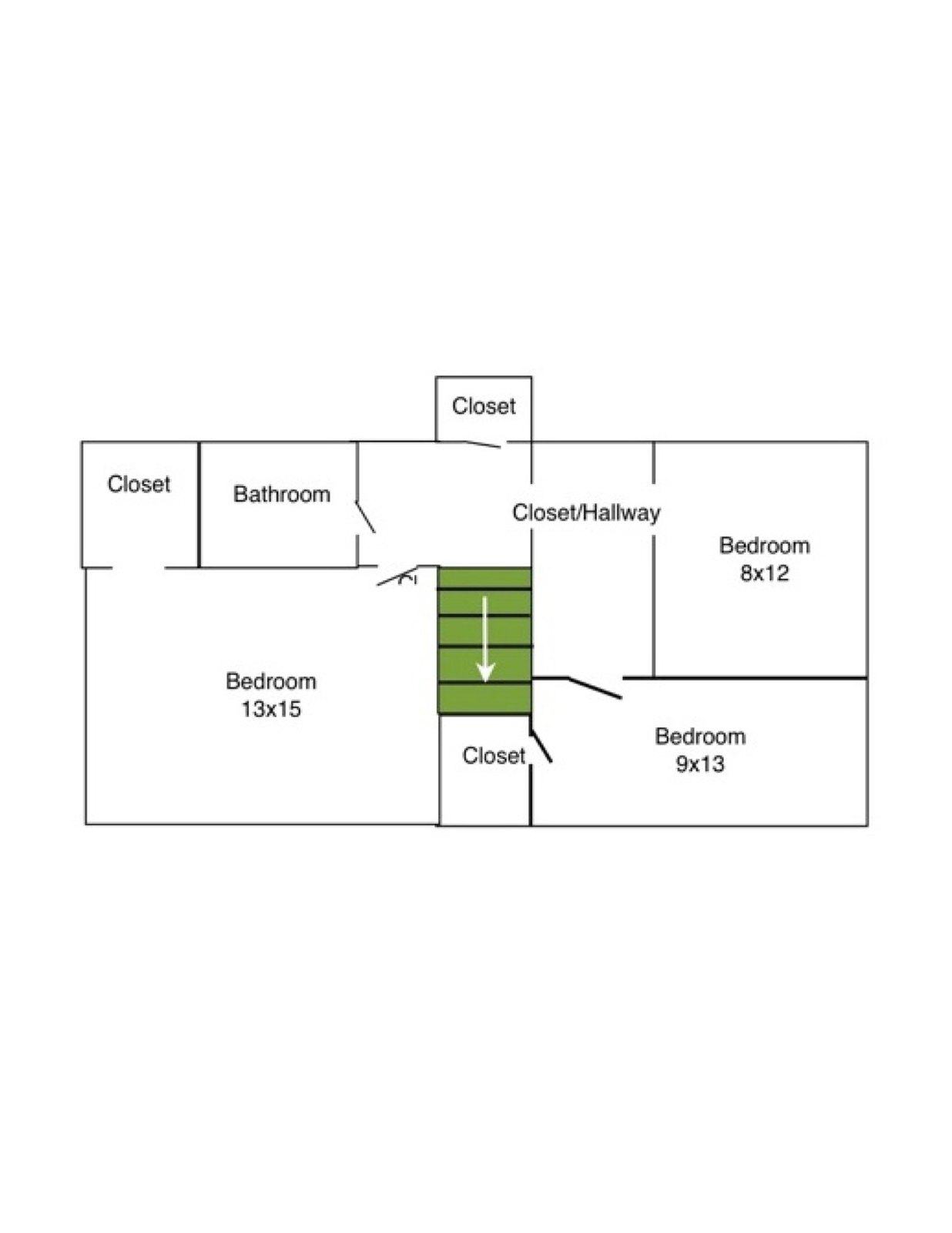The detailed floor plan, outlined in blue, showcases the upper floor of a spacious apartment or house. At the top of the layout, there is a small closet. On the left side, a sequence of rooms begins with a closet, followed by a bathroom, and then a sizable bedroom measuring 13 by 15 feet. This bedroom has a door that opens into a hallway, with the top-positioned closet adjacent to it.

Beneath this hallway, green-colored steps descend into another closet space. The words "closet hallway" are visibly marked in blue lettering within the plan. Next to this area, there is a bedroom measuring 8 by 12 feet, followed by a third bedroom that measures 9 by 13 feet.

In summary, the upper floor includes three bedrooms—one large and two smaller ones—a bathroom, and multiple closets, all arranged in a well-structured and functional layout.